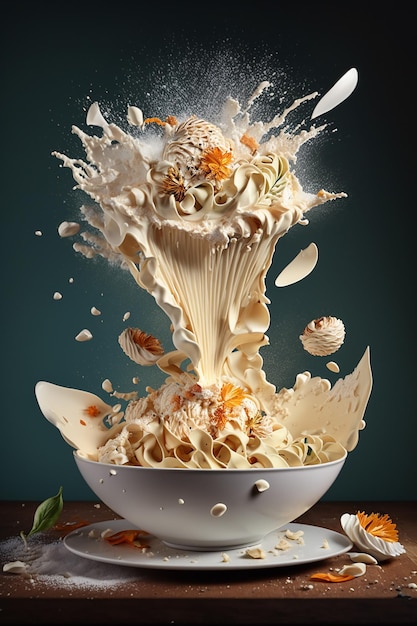In this vertically rectangular, digitally produced, full-color photograph taken indoors with artificial lighting, an artistic and visually striking scene is depicted. The composition primarily features a brown wooden countertop or table at the base with a white dish and bowl positioned on it. Behind the setup is a dark blue wall that enhances the contrast of the objects in the foreground. Central to the image is a white, creamy substance that looks like a dramatic splash captured in mid-air, giving the impression something big has been dropped into the bowl. This splash is highly textured and filled with geometric shapes including ovals and vertical lines, some resembling horns, adding an artificial and meticulously crafted feel to the visual. The white substance, possibly resembling ice cream or flowers, includes elements with frosting colors and little orange bits, making it appear both edible and abstract. Additionally, a pile of sugar, a green leaf, and another white element are subtly placed on the table, further adding to the intricate details of this artistically posed image.